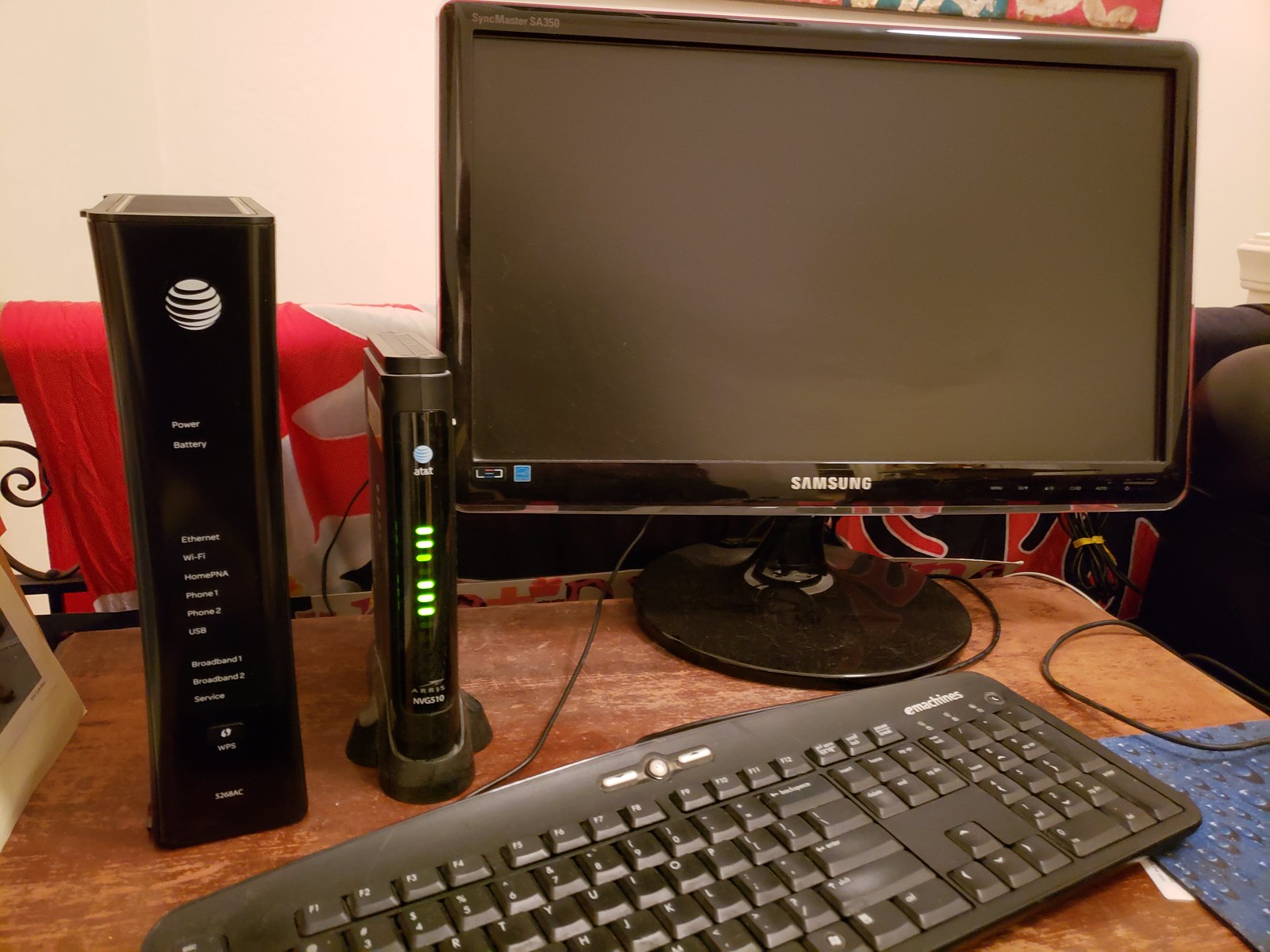This color photograph captures a detailed view of a home office setup. Dominating the wooden tabletop is a sleek black Samsung monitor with a clear frame accent and circular base, prominently displaying the branded 'Samsung' logo. In front of the monitor sits a black keyboard paired with a dark blue mouse pad, designed with opaque raindrop patterns set against its blue background. To the left, a silver-framed LCD clock is partially visible, suggesting meticulous attention to timekeeping in this workspace.

Alongside the monitor on the right, two AT&T modems are positioned. The larger modem sports an array of lights and labels, including "Power," "Battery," "Ethernet," "Wi-Fi," "Home," "PNA," "Phone 1," "Phone 2," "USB," "Broadband 1," "Broadband 2," "Service," followed by a 'WPS' button and the model number '5268AC'. The smaller modem features the AT&T logo in light blue, accompanied by several green indicator lights and the label 'NVG S10'. Together, these elements suggest a robust internet setup.

To the left of the desk, a chair draped in a red and white sheet adds a touch of casual comfort to the workspace. The harmonious placement of technology and personal touches offers a glimpse into a functional and personalized home office environment.